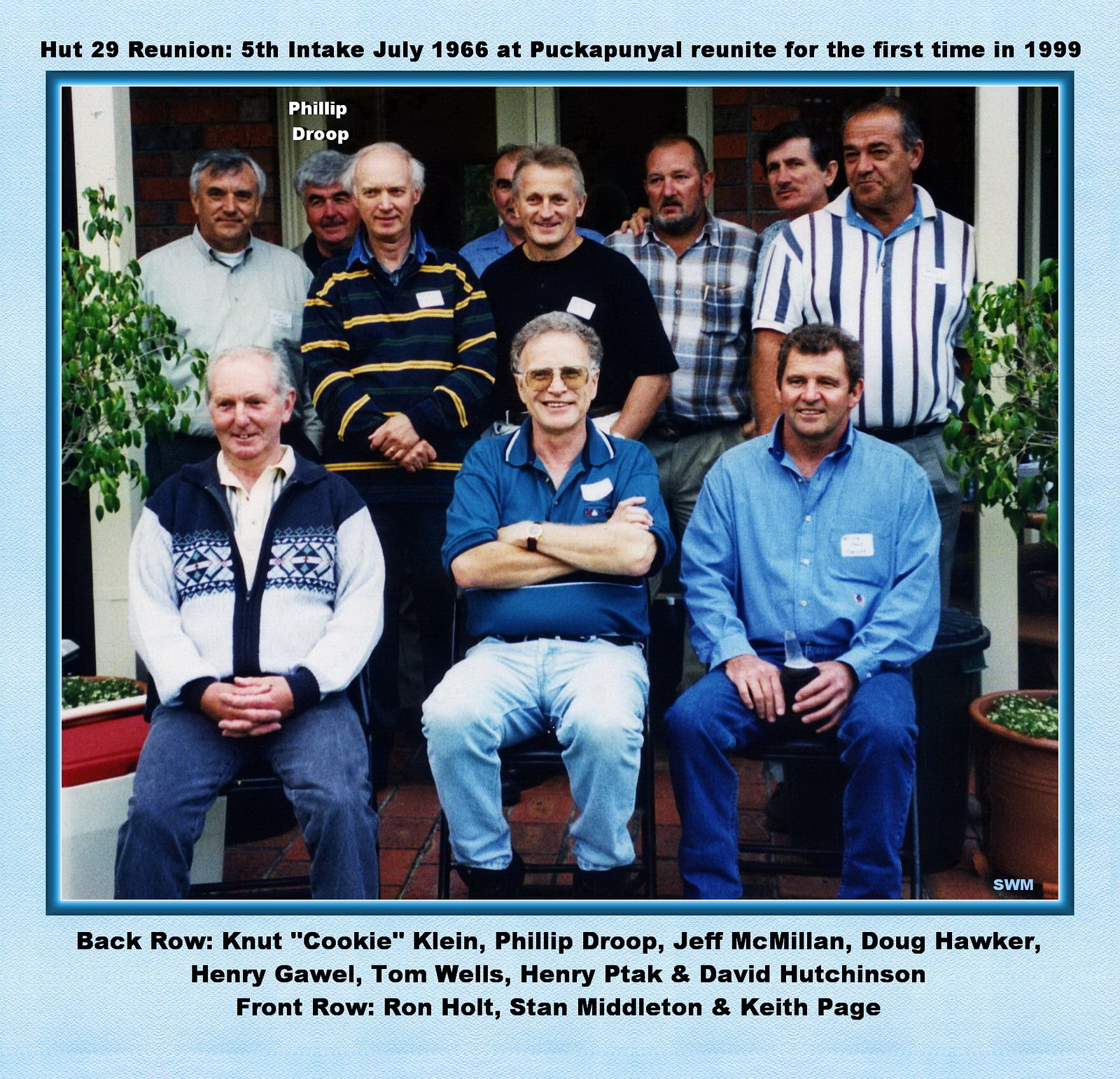The photograph features a group of eleven men with a blue border approximately half an inch thick on the left, top, and right sides, and about an inch at the bottom. There are three men seated in the front row and eight men standing in the back row. Notably, the man second from the left in the back row is identified as Philip Droop in small white text. The individuals in the back row are listed with names from left to right: Ned Cookey-Klein, Phillip Droop, Beth Different-Whelan, Doug Hawker, Henry Getwell, Tom Wills, Henry Tack, and David Hutchinson. The front row consists of Ron Holt, Stan Middleton, and Keith Page. The man in the middle of the front row wears sunglasses, a blue collared shirt, and lighter blue jeans, while the man to his right has dark hair, no glasses, a blue button-up shirt, and blue jeans, holding a beverage. The man on the left of the front row wears a sweater and blue jeans. Around the edges of the image, small plant leaves are visible. The caption at the top reads: “Hut 29 reunion, 5th intake, July 1966 at Pokoponyo. Reunites for the first time in 1999.” The overall image seems to commemorate medical volunteers, possibly those who served in Vietnam, with names listed below each individual.